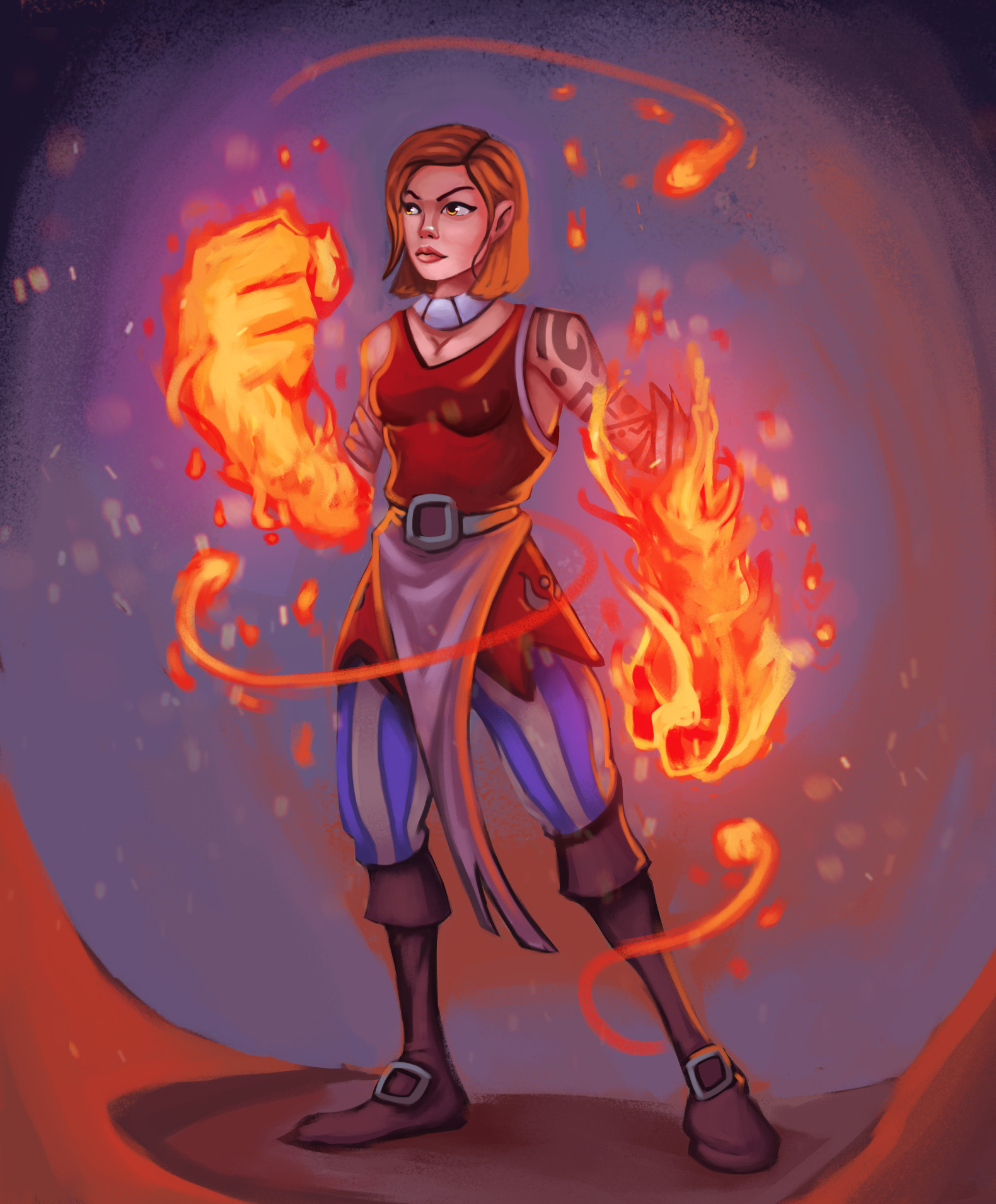The image is a highly detailed, cartoon-like illustration of a determined-looking woman with magical powers. She stands in an indistinct area with a swirling blue and orange background, and she's positioned on a darker surface with an orange layer beneath it. The woman has vibrant red hair cut just above her shoulders and fair skin. 

She's dressed in a sleeveless, ripped red tunic that reveals her bra underneath. The tunic, which ends at her thighs, is overlain by an additional skirt-like garment. She wears a silver necklace and a belt around her waist, coupled with puffy blue and white striped pants tucked into knee-high brown boots with square, metallic silver buckles. Her exposed arms are adorned with black tattoos in spiral and geometric patterns.

Both of her arms, from her hands up to her elbows, are encased in bright, vibrant flames, producing much larger, flaming fists—evident she possesses a powerful and fiery superpower. Wisps of flame and sparks encircle her, creating an animated atmosphere, with one wisp above her head, one around her waist, and another around her right leg. 

This painting captures a dynamic and mystical scene, blending elements of fantasy and cartoon artistry.